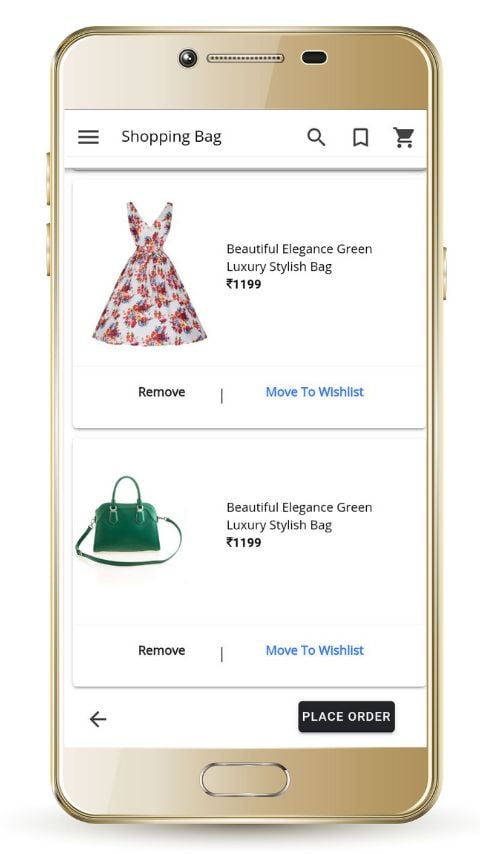A luxurious green purse, priced at $1,199, stands elegantly in a vibrant setting adorned with flowers. The stylish bag, a highlight of the scene, is prominently featured alongside a shopping cart and a white dress. The interface displays various options such as "Remove," "Move to Wish List," and "Place Order," with the price "1,199" in bold black text. "Move to Wish List" is distinctly written in blue, while other options are in black. 

Next to the shopping details is a sleek gold smartphone with a silver-bordered home button, showing a detailed viewport of an online shopping app. The phone, presenting volume keys on the top left, a power button towards the top right, a speaker in the top middle, and a camera with a black sensor, possibly IR sensor, to the left.